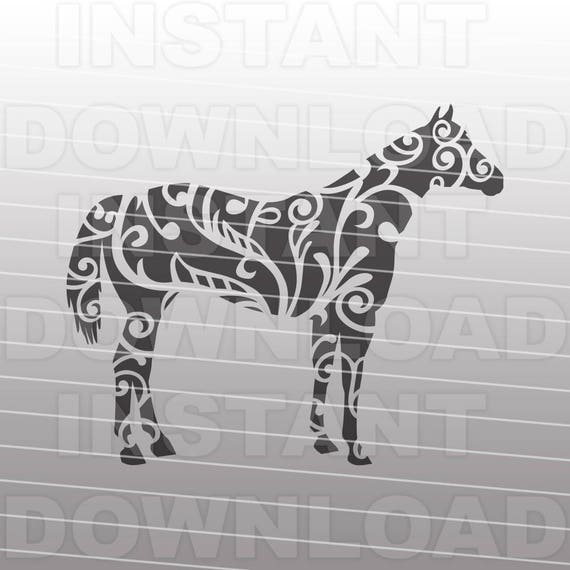This is a large square, black, white, and gray vector graphic image with no border. The image prominently features a decorative, side-profile silhouette of a horse facing right. The horse, shaded in black and dark gray, is adorned with intricate white filigree and leaf patterns, emphasizing its elegant form. The background is a gradient that transitions from almost white at the top to dark gray at the bottom. White, slightly diagonal lines stretch across the image from the upper left to the right. The phrase "instant download" is repeatedly watermarked across the entire background in large white block letters, starting from the top and continuing downwards.